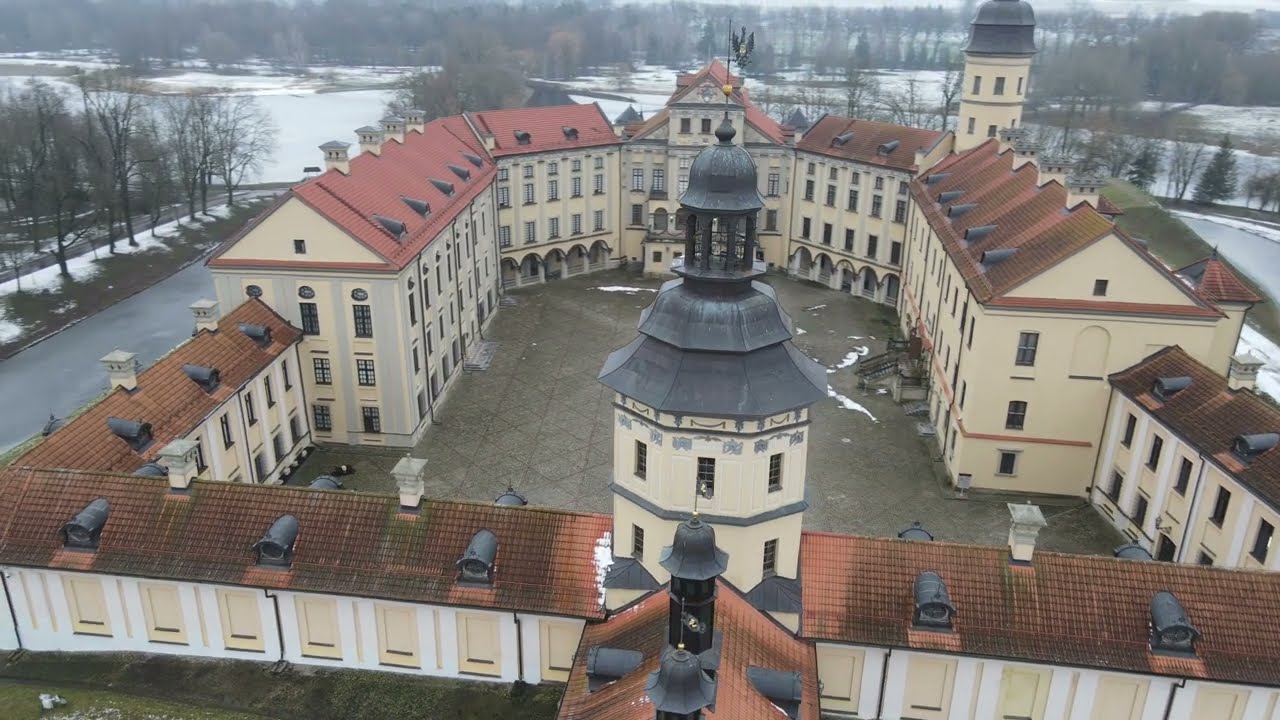The aerial photograph depicts a large, symmetrically designed building complex that could be a church, school, or college. The tan-colored structure, possibly made of concrete or brick, features two prominent towers—one in the front middle and another in the back right—each roughly three stories taller than the rest of the three-story building. The building has a distinctive red or maroon roof and encircles a gray cement courtyard, accessible by black steps. Surrounding the building are clear streets devoid of cars or people, with fields and trees extending into the background, all dusted with snow under an overcast sky. Farther away, there's a small pond or lake and a density of leafless trees, enhancing the cold, serene atmosphere. The entire area has a quaint, homey charm, resembling a small village or university setting.